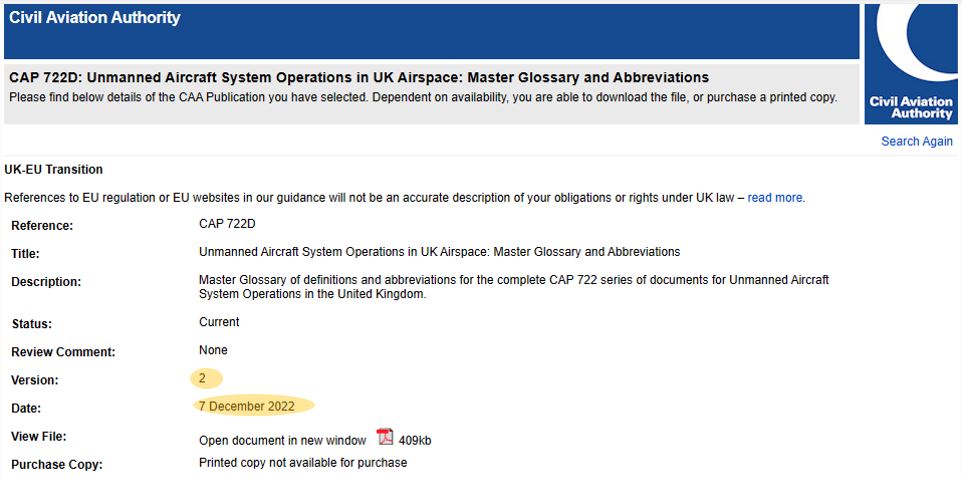The image features a structured layout that begins with a dark blue border at the top. This border contains white text that reads "Civil Aviation Authority." Directly beneath this is a light gray box of a similar size, which features black text. The text reads, "CAP-72-2D: Unmanned Aircraft System Operation in UK Airspace: Master Glossary and Abbreviation." 

Below this, in smaller text, it states, "Please find below details of the CAA publication you have selected. Depending on availability, you're able to download the file or purchase a printed copy."

To the right, there is a dark blue box, matching the color of the top border. This box is approximately an inch wide and extends the combined height of both the blue border and the gray box. Through the center of this dark blue box runs a curved white line. Beneath the line, white text reads "Civil Aviation Authority." Following this, there is a blue hyperlink labeled "Search Again." 

At the bottom of the image, a light gray line spans the entire width, connecting the left and right edges.